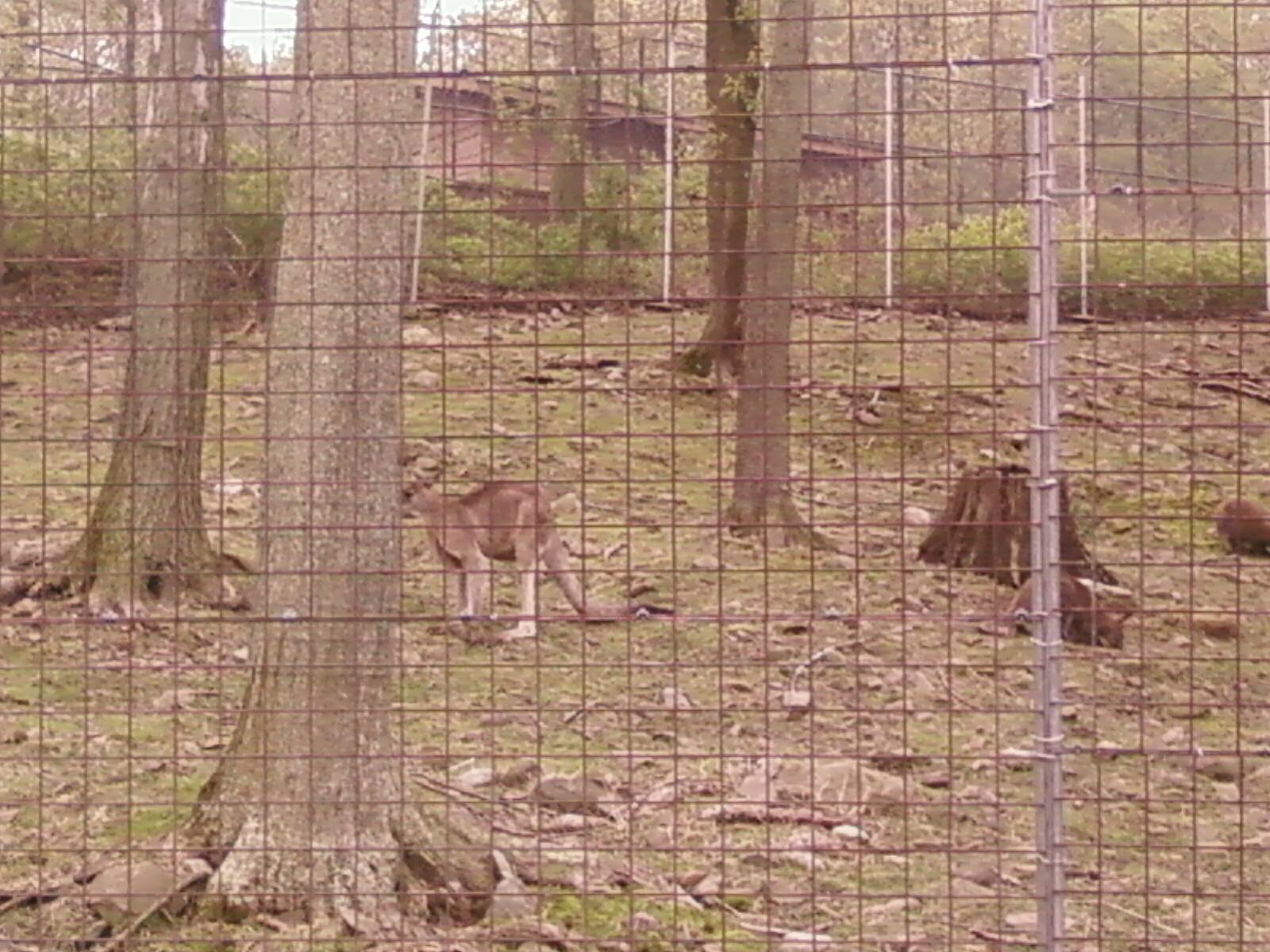In the photograph, a solitary kangaroo stands on its hind legs in the middle of a enclosed pen situated on a gradual hillside. The scene is encased in a tall, approximately 15-feet-high metal fence composed of crisscrossed wires forming small squares that are about two to three inches wide, sufficient to prevent the kangaroo from escaping. The pen features a captivating mix of natural and man-made elements: there are four tall tree trunks, some visibly located on the left side, and a scattering of gray-brown wooden pieces and rocks across the ground. In the foreground, tall steel poles support the fence, and a gate is positioned near where the photo was taken.

The pen is nestled in a small grove of trees, providing a shaded and secluded environment for the kangaroo. To the right side of the picture, two small furry creatures can be seen, potentially miniature kangaroos, alongside a tree stump. In the background, on top of the hill, a series of shrubs and another fence lead up to a large brown building that resembles a house or office. Beyond this building, a dense forest of trees frames the scene, further enriching the photograph with layers of natural beauty and human intervention.